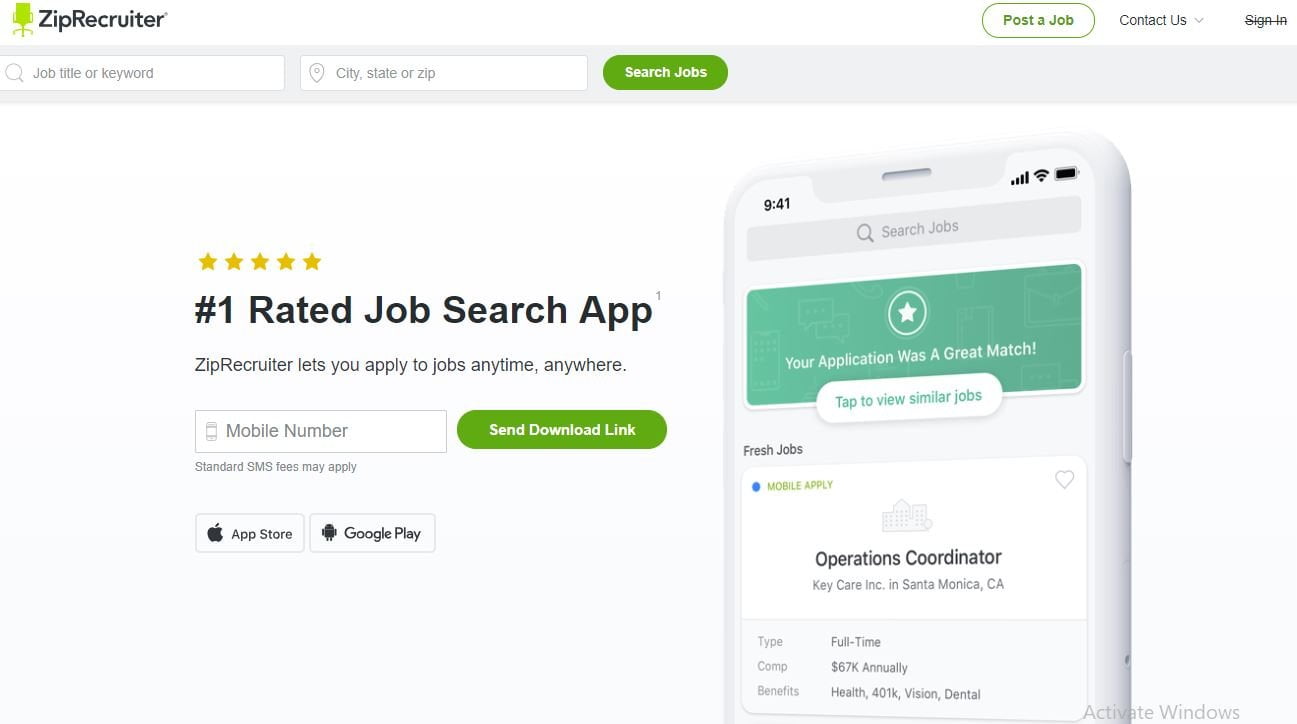This screenshot captures the homepage of the ZipRecruiter website, characterized by its clean, white background. In the upper left corner, the ZipRecruiter logo is prominently displayed. The logo features "ZipRecruiter" written in black font with "ZIP" and "R" capitalized, and includes a small green office chair icon to the left.

Below the logo, the top navigation menu is visible, featuring a white search box set against a very light gray background. The search box includes two rectangular input fields: the first prompts for a job title or keyword, and the second for a city, state, or zip code. Adjacent to the input fields is a green search button with rounded corners and "Search Jobs" written in white font.

Dominating the main section of the website is a bold headline in black font that reads "Number 1 Rated Job Search App." Above this headline are five gold stars, denoting high ratings. The text below the headline explains that "ZipRecruiter lets you apply to jobs anywhere, anytime." Directly under this description, there is a field prompting users to enter their mobile number, followed by a green button labeled "Send Download Link."

To the right, there is a graphical illustration of a smartphone displaying the ZipRecruiter app interface. The app screen showcases a message at the top stating, "Your application was a great match."